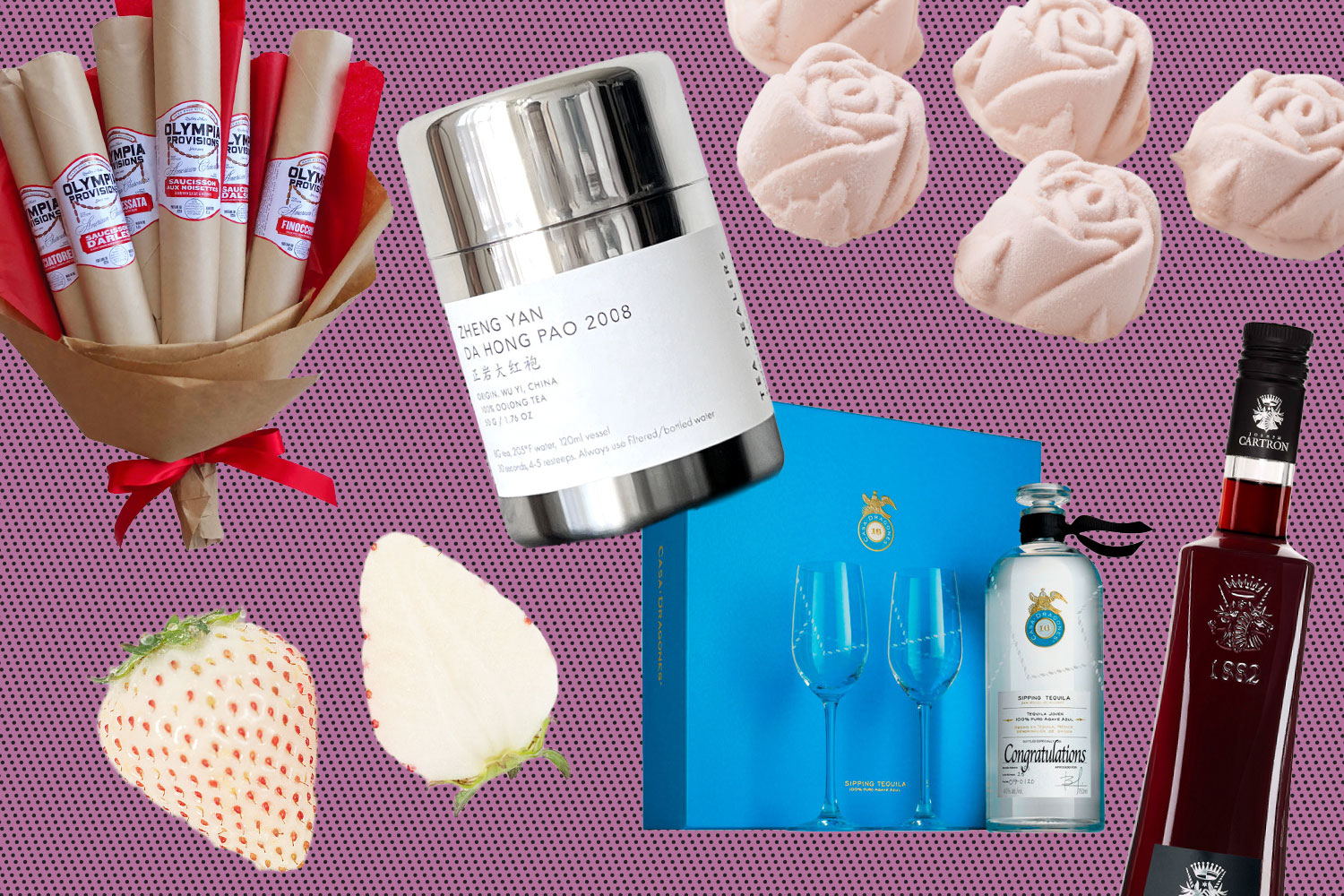The image presents a digitally composed scene with various products arranged against a mauve mesh background. Starting from the bottom left corner, there is a white strawberry cut in half, displaying its unique white flesh and red polka dot seeds, topped with a green leaf. Above this is a small basket wrapped in craft paper labeled "Olympia Provisions," containing several cylindrical items, possibly cigars or salami. To the right of the basket, a silver thermos with a white label reading "Jingyan Dahongpao 2008" in both Asian characters and English is prominently featured. Continuing clockwise, a cluster of what appear to be either white candies or folded white towels is placed above a bottle that could contain either olive oil or red vinegar. In the lower right corner, there is a distinctive tall, dark brown bottle labeled "Cartron," featuring a crown, two unicorns, and the number "1882." Adjacent to this, a blue box is shown containing a set that includes two glass flutes and a liqueur bottle, with "Congratulations" visibly inscribed on the decanter. Each item is meticulously cut out and layered onto the composite, creating an intriguing and detailed visual narrative.